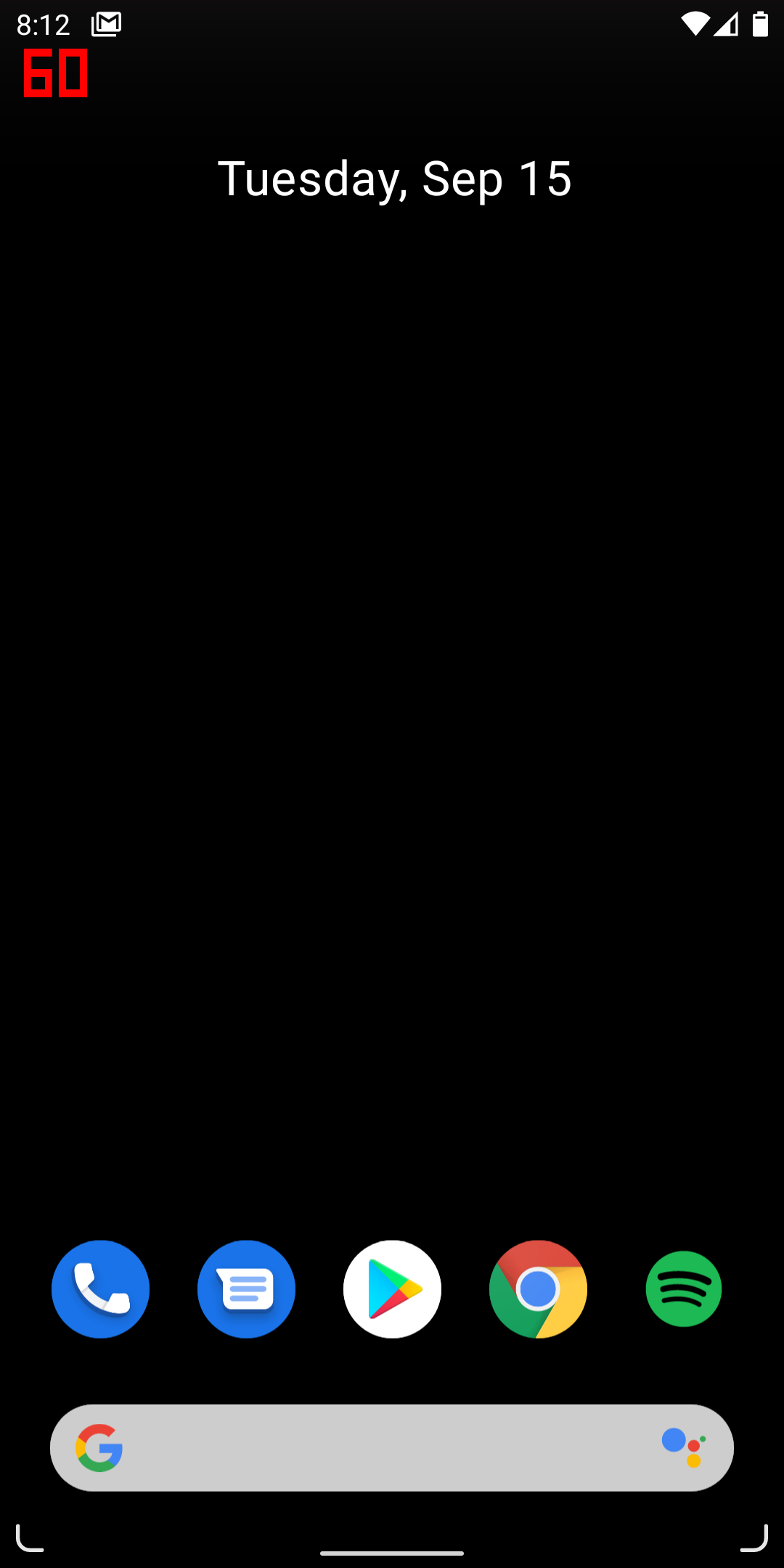The image appears to be a screenshot from an Android device, characterized by its rectangular shape. At the very top of the screen, the time is displayed as 8:12. To the right of the time, there is a small notification icon, likely indicating an email, possibly from the Gmail app. Additionally, there are three familiar icons on the right side: a Wi-Fi icon, a cellular signal bar that is three-quarters full, and a battery icon that shows almost full charge.

The date is prominently displayed in the top center of the screen in white text, reading "Tuesday, September 15th." The background of the entire screen is black, functioning as a screensaver. At the very bottom of the screen, there is a Google search bar featuring the multicolored 'G' logo (red, yellow, green, and blue) and the Google Assistant symbol.

Aligned at the bottom are five app icons: 
1. A blue and white icon for the phone app,
2. A blue and white icon for text messages,
3. A white icon with a multicolored triangle representing the Google Play Store,
4. The Chrome browser icon, which is a red, green, and yellow circle with a blue and white center,
5. The Spotify app icon, which is green and black.